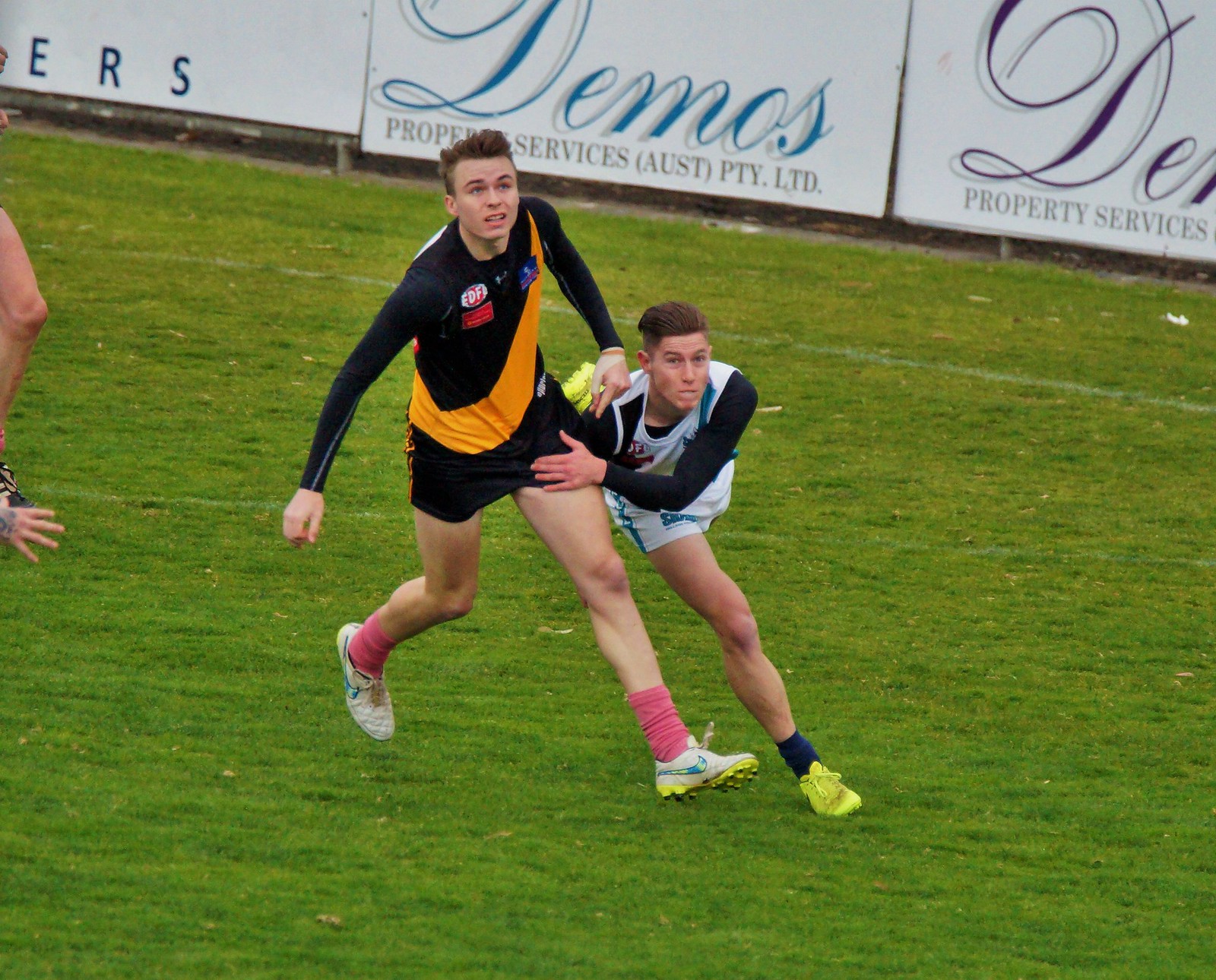In this vibrant outdoor photo of a soccer match, two players are captured in mid-action as they sprint across a lush green field. The player on the left, tall and athletic, wears a black long-sleeve jersey adorned with an orange stripe, complemented by black shorts, pink socks, and white Nike shoes featuring a rainbow swoosh. His opponent, positioned to the right, appears to be in the midst of stumbling, reaching out to grasp the tall player’s thigh, possibly to steady himself. This opponent is clad in a white jersey with black long sleeves, white shorts, and blue socks. The backdrop features signage with words like "demos" and "property services," adding context to the scene. Additionally, just off to the left edge of the frame, a hand and part of a leg are faintly visible, hinting at the presence of another player on the field.